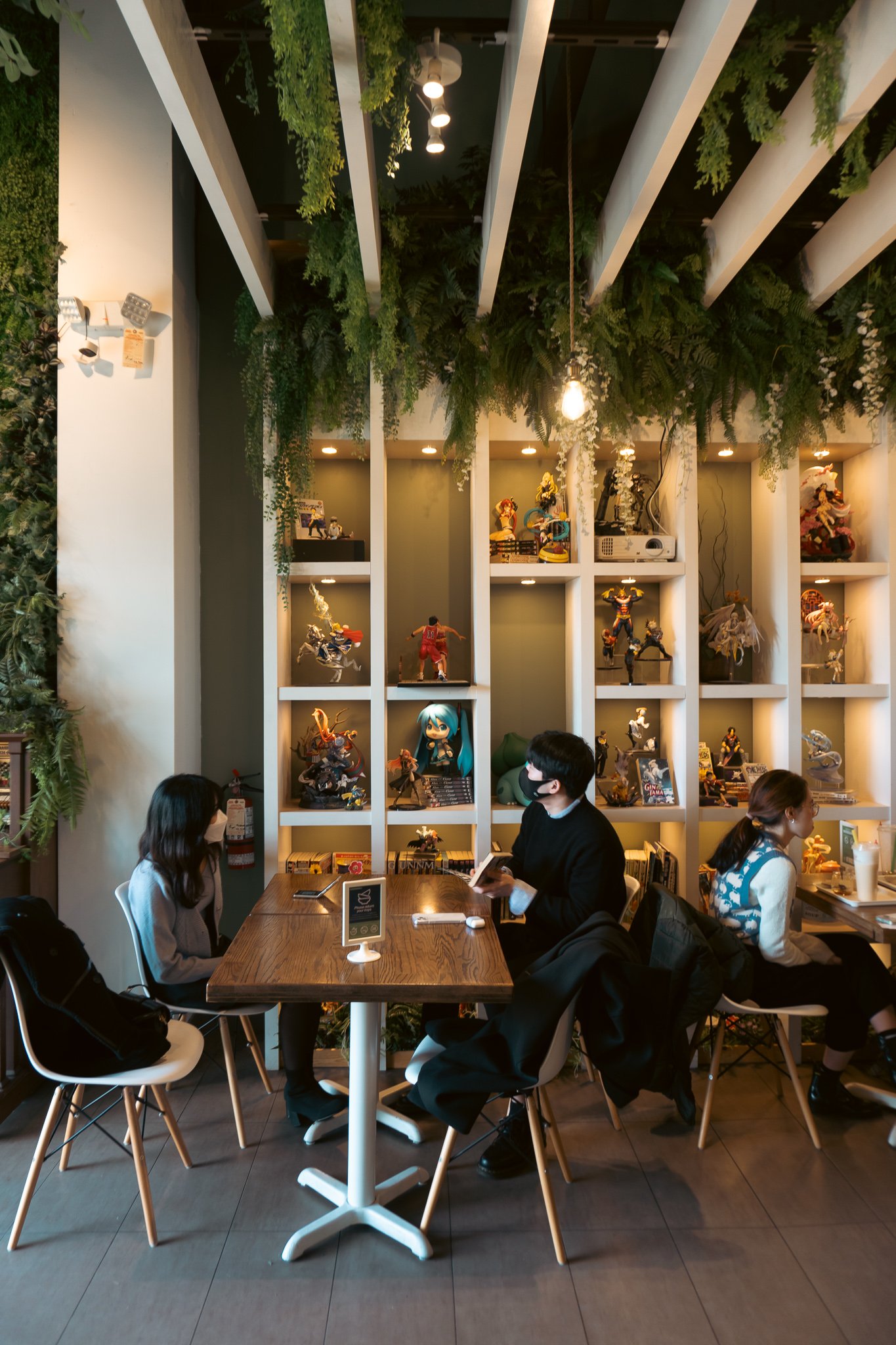In this image, a couple is seated at a wooden table in a uniquely decorated restaurant or coffee shop, each wearing face masks. They share the space with a woman on the right, who is also sitting at a separate table, dressed in a blue sweater, white blouse, and black pants. The table they are seated at has a white base with an X-shaped design, set against a wood floor, and holds a menu along with a woman's backpack occupying a nearby seat. The backdrop features a white shelf filled with intricately lit figurines, including sports figures, fantasy figures, and dolls, suggestive of an anime or Japanese theme. The shelf is segmented into box-like areas, each illuminated to showcase the detailed models. Above the diners, white slat boards with green foliage hanging down create a cozy atmosphere, complemented by a rope-held light bulb dangling from the ceiling. The woman on the right does not wear a mask and is turned away from the couple seated at the table.